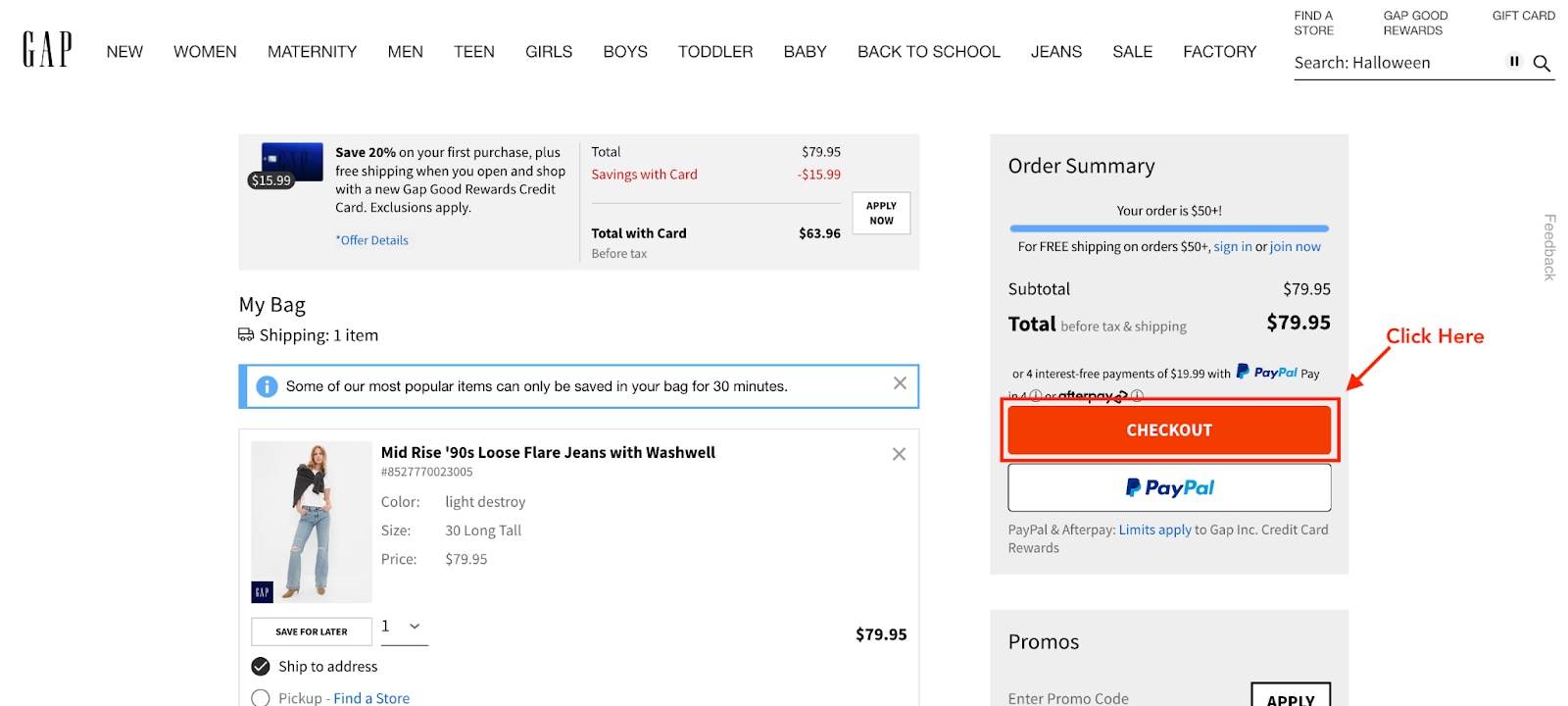The image depicts a screenshot of the Gap website. At the top, there's a navigation bar featuring categories such as New, Women, Maternity, Men, Teen, Girls, Boys, Toddlers, Baby, Back to School, Jeans, Sale, and Factory. On the upper right-hand corner, the subcategories include options like Find a Store, Gap Good Rewards, and a search function, all in capital letters. Next to the search bar is a magnifying glass icon.

Below the navigation bar, there's a prominent rectangular banner on the left side displaying a promotional offer. The banner reads: "$15.99 - Save 20% on your first purchase, plus free shipping when you shop with a new Gap Good Rewards credit card. Exclusions apply. Offer details." This text is highlighted in blue. The banner also provides a breakdown of the shopping total: the original total is $79.95, resulting savings with the card is $15.99, leading to a new total of $63.96. An "Apply Now" button is also present.

Below this promotional banner, there's a section titled "My Bag" showing one item. It notes that some popular items can only be saved in the shopping bag for 30 minutes. The item listed is "Mid-Rise 90s Loose Flare Jeans with Washwell," showing details such as color, size, and price ($79.95).

On the right side of the page, the order summary is displayed in gray, with a red "Checkout" button featuring an arrow icon. Below this button is an option to check out with PayPal.